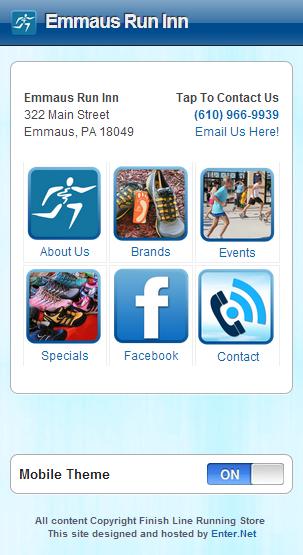This is a vertical rectangular screenshot from the app "eMouse Run In" displayed on a mobile device. At the top, there is a dark blue band featuring the title, "eMouse Run In," along with its address, 322 Main Street, Emmaus, Pennsylvania, 18049. The opposite side of the top band provides a clickable phone number, 610-966-9939, and an "Email Us Here" link for contacting the store.

Below the top band, a white rectangle displays six icons or widgets labeled About Us, Brands, Events, Specials, Facebook, and Contact. These widgets allow users to navigate to various sections of the app. The background beneath the white panel is light blue, contrasting with the dark blue top.

At the bottom of the screenshot, there's a toggle button indicating that the mobile theme is currently on. Further down, copyright information reads, "All content, copyright Finish Line Running Store." The overall color scheme alternates between dark blue, light blue, and white, providing a clean, organized layout for easy navigation.